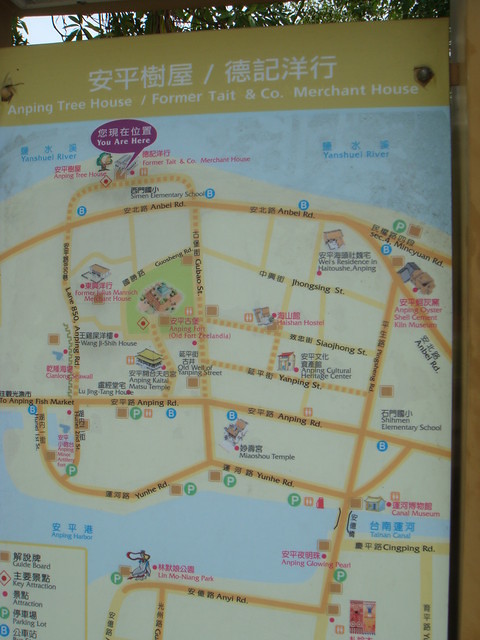This photograph showcases a detailed map, prominently featuring the "Anping Treehouse / Former Tate and Company Merchant House." At the top of the map, Chinese characters in white are displayed against a goldish-yellow background, followed by the English translation beneath. The map itself is set against a blue background and illustrates various streets marked with dashed and solid yellow lines, naming the roads and key locations. Points of interest, including parking lots and possibly restaurants, are highlighted. Two bodies of water flank the land on either side, with additional water elements depicted at the bottom. The map includes a legend in both Chinese and English, providing icons and explanations for different types of points of interest, making it a comprehensive guide to the local area.